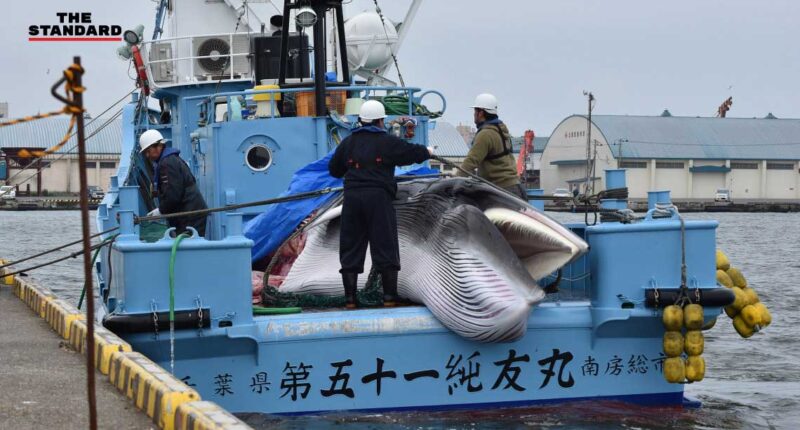A teal blue Chinese fishing boat is docked near a concrete platform. The boat, identified by the kanji characters on its hull, features a flatbed area where three men stand. These men, donned in white hard hats and work attire - one in a long-sleeve brown sweatshirt, another in black overalls, and the third in a dark jacket, are engaged in handling a large black and white whale. The whale's mouth is slightly agape, exposing a pink and fleshy interior beneath a blue tarp covering its body. One man at the center, with his face not visible, appears to be positioning a tool inside the whale's mouth. To his right, another man in green assists in dragging the whale onto the boat. On the far left, a man with his face partially visible is observed looking at something on the boat. In the background, a building with an arched top and several garage doors can be seen, and the partly cloudy sky adds a bluish hue to the scene. Additional yellow objects or tools hang from the side of the boat, enhancing the work setting atmosphere.